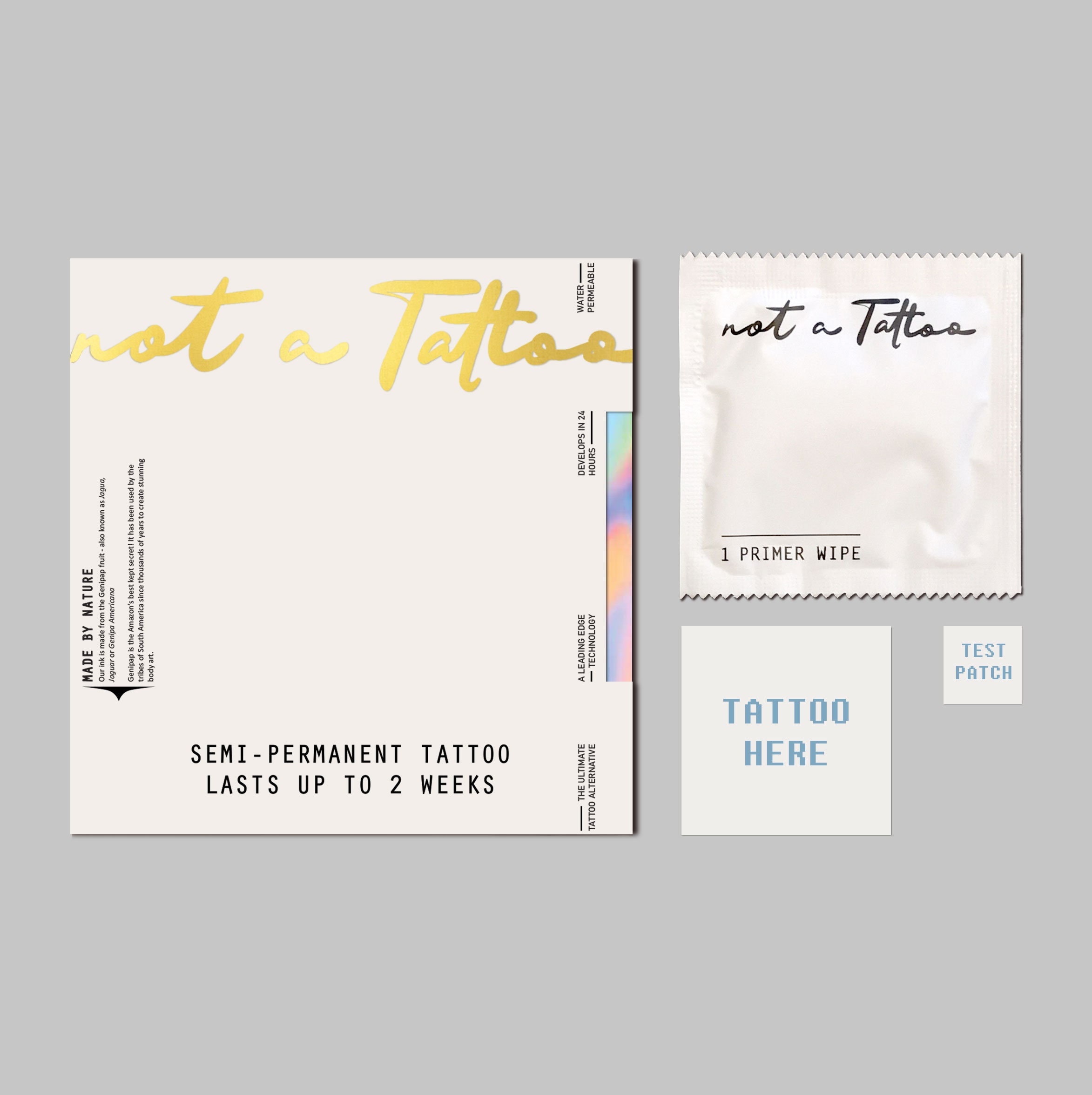In the close-up photograph, several paper objects are neatly arranged on a grey background. The main focus is on a square piece of paper on the left-hand side. This piece has a gold cursive inscription at the top that reads “Not a tattoo,” where the cursive appears reflective under the light. Below this, at the bottom of the square, black text states, “Semi-permanent tattoo, lasts up to two weeks.” Directly to the right, there's a slightly larger white envelope with frilled edges containing a primer wipe. This packet has black text at the bottom-left corner that says, “1. Primer wipe,” and also features the repeated cursive phrase “Not a tattoo.” Below this envelope is a small white square labeled “Tattoo here” in blue, and to the right of this square is another slightly smaller square that reads “Test Patch,” also in blue. Together, these elements form a detailed collection of items related to semi-permanent tattoos, emphasizing their non-permanent nature and the preparatory wipes included.